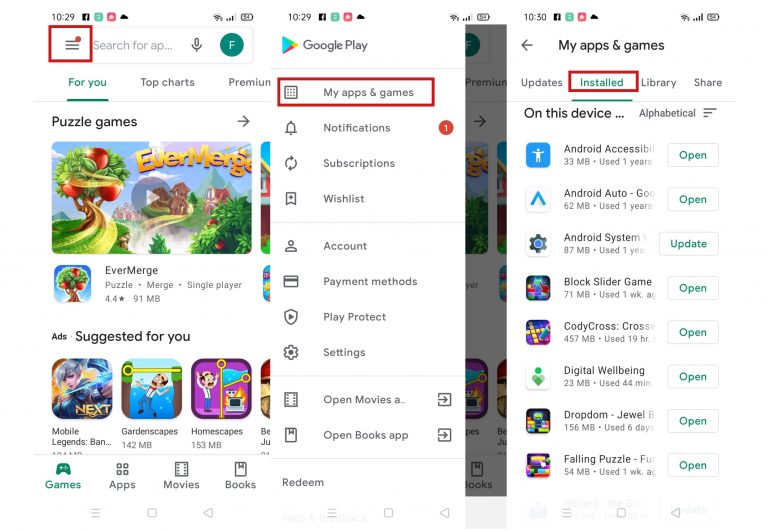The image is divided into three sections, each highlighting a different feature of the Play Store application on a smartphone.

**Left Section:** The focus is on the main Play Store page. The top-left corner features a red outline around the notification icon. Below that, there's a search bar with the tabs "For You," "Top Charts," and "Premium" visible. The highlighted game is "EverMatch," a 91MB puzzle game. The game display includes vibrant graphics with yellow backgrounds, green trees, and red fruits. Below it, suggested games include "Mobile Legends," "Gardenscapes," and "Homescapes." At the bottom, navigation buttons for "Games," "Apps," "Movies," and "Books" are shown, with the "Games" tab currently selected and highlighted in green.

**Center Section:** This section features the Play Store menu drawer, opened and highlighted with a red outline around the "My Apps and Games" option. The menu items listed below include "Notifications" (showing one notification), "Subscriptions," "Wishlist," "Account," "Payment Methods," "Play Protect," "Settings," "Open Movies App," "Open Books App," and a "Return" option at the bottom.

**Right Section:** The "My Apps and Games" menu is fully opened, showing options like "Update," "Installed," "Library," and "Share" at the top. The "Installed" tab is highlighted in blue. Below, a list of installed applications is presented, featuring "Android Accessibility," "Android Auto," and "Android System" (with an update button in green). Other apps listed include "Block Slider Game," "CodeCross," "Digital Whirlpool," "Drop Dome," and "Falling Puzzle," with most having an "Open" button next to them, aside from those needing updates.